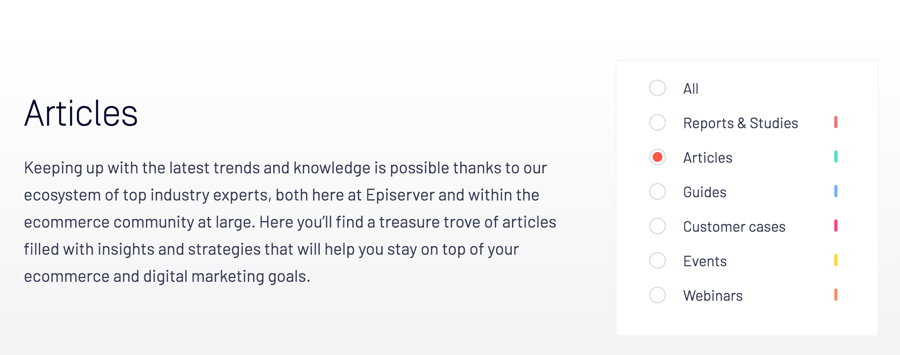The image showcases a white background with black text and several elements divided into two sections. On the left, there is a prominent headline in large font, accompanied by a paragraph below. The paragraph reads: "Keeping up with the latest trends and knowledge is possible, thanks to our ecosystem of top industry experts, both here at EpiServer and within the e-commerce community at large. We hope you'll find a treasure trove of articles filled with insights and strategies that will help you stay on top of your e-commerce and digital marketing goals."

To the right, there is a panel in a lighter shade, featuring a vertical sequence of colored bubbles, each adjacent to specific categories. The topmost bubble is labeled "All" with black text. Following that, a bubble labeled "Reports and Studies" has a red mark beside it. The "Articles" section is highlighted with a red bubble. The "Guides" category is marked with a green color, while "Customer Cases" is annotated in blue. "Events" has a yellow highlight, and "Webinars" is marked with red. This detailed arrangement categorizes the different types of content available, providing a streamlined navigation system for users.